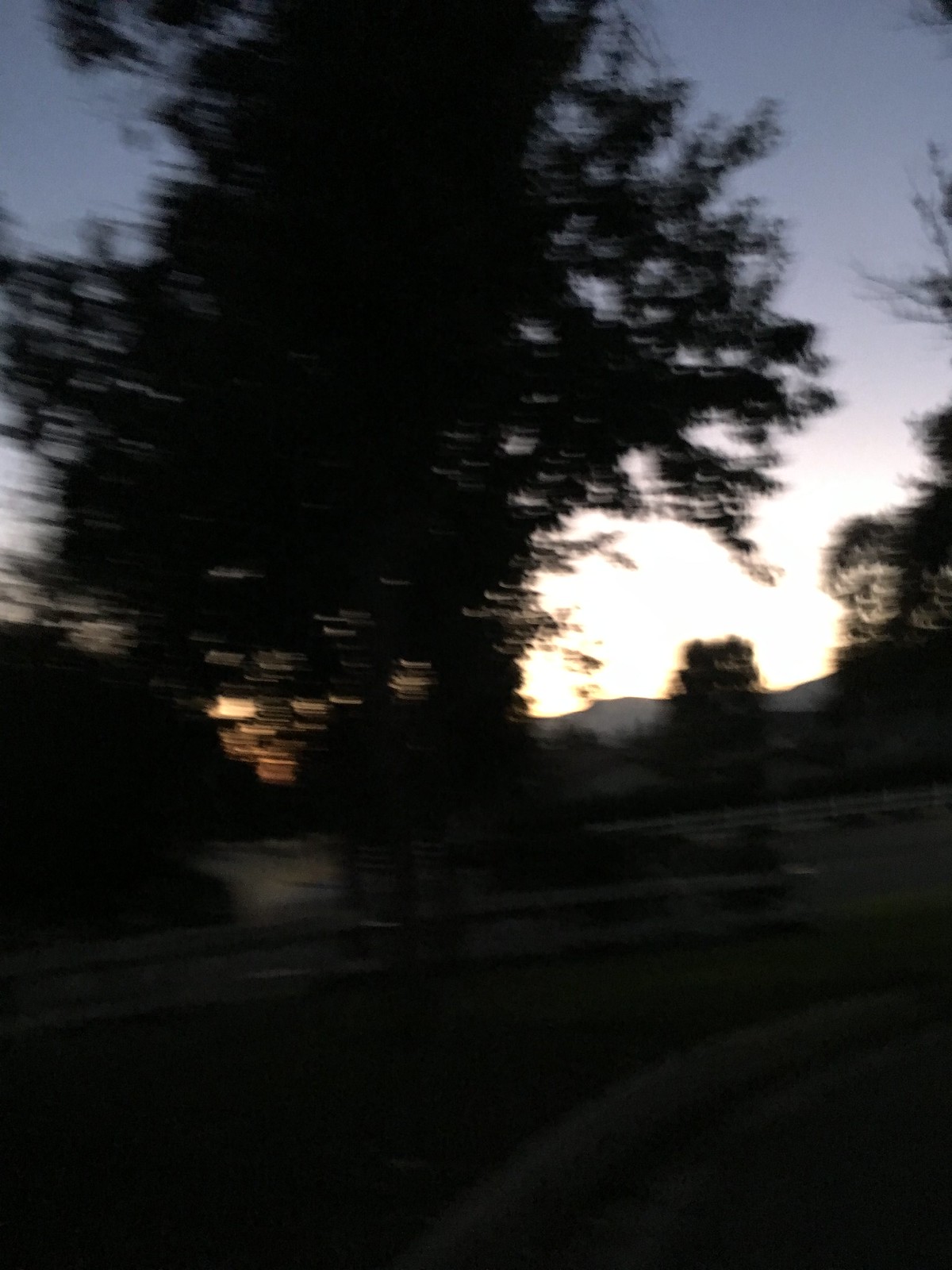A blurry photograph captures an evening scene of the outdoors. Dominating the image is a lone tree cloaked in the dim light of dusk, nestled in shadow. The majority of the background presents a nondescript, light gray overcast, indicative of the sun retreating for the day. Partial illumination suggests a setting sun positioned obscurely behind the tree, casting subtle, uneven transitions of light around its center but not reaching its upper branches. The indistinct focus renders the colors ambiguous, accentuating the mysterious, transient nature of twilight.